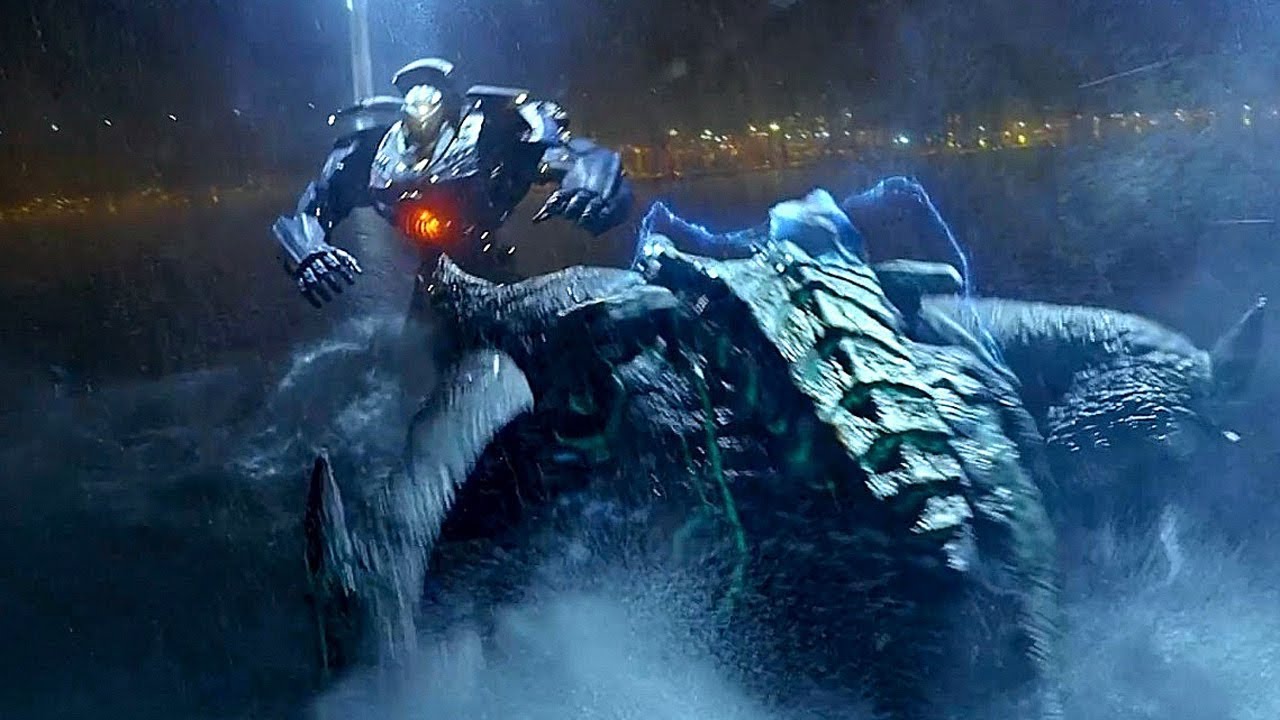In this blurred, cinematic image from the movie *Pacific Rim*, a large alien monster and a giant robot are locked in battle in what seems to be the middle of a large body of water, possibly the ocean. The monster, with its back to the camera, displays large green and black scales, visible green vessels along its back, and blue tentacles protruding from its head. The robot, on the other hand, faces both the monster and the camera, showcasing its blue and silver plating and a glowing red power core on its chest. The dramatic scene is set against a night-time city skyline, with the lights of distant buildings twinkling in the background, enhancing the sci-fi atmosphere of the showdown.